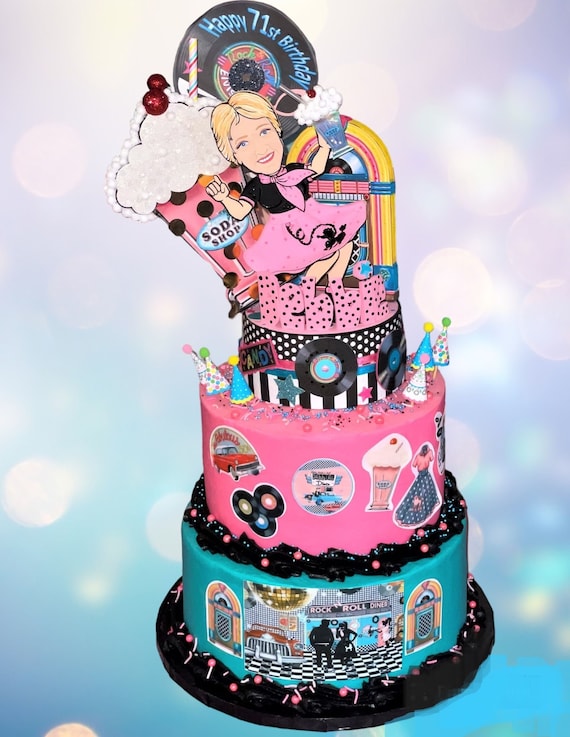This vibrant and visually captivating three-tiered birthday cake is crafted for a 71st birthday celebration with a nostalgic 1950s rock-and-roll soda shop theme. The bottom layer is adorned in blue fondant and features intricate black and white images of iconic jukeboxes, a classic red car, and a lively rock-and-roll diner scene complete with a black and white checkerboard floor and a couple dancing beneath a gold disco ball. Ascending to the second tier, the hot pink fondant layer showcases whimsical 50s imagery, including three vinyl records, a sparkling ice cream soda topped with whipped cream and a cherry, a red car, and decorative motifs of poodle skirts and kitten sweaters. The top black and white striped layer is embellished with miniature vinyl records and party hats. Crowning the cake is a figurine of the birthday celebrant, elegantly dressed in a 50s-style pink skirt, black top, matching sweater, and pink handkerchief around her neck, holding an ice cream float beside a large jukebox and a vinyl record that reads "Happy 71st Birthday." This cake masterfully encapsulates the vibrant energy and nostalgic charm of a 1950s sock hop, making it a stunning centerpiece for the birthday bash.